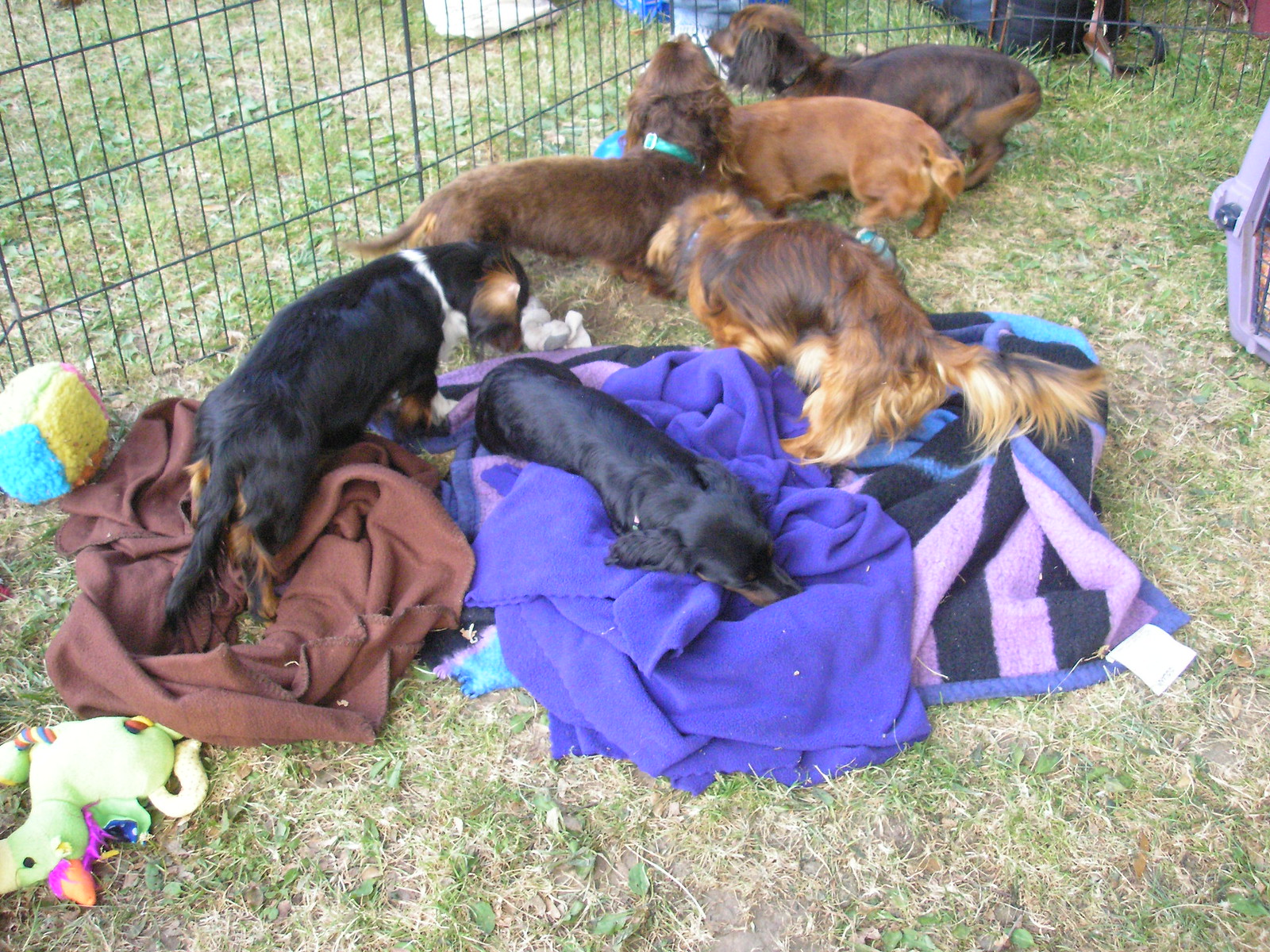This detailed color photograph captures an outdoor scene set in a grassy field, possibly at a dog show or adoption event. Within a chicken wire-like fenced enclosure, six medium-sized dogs of the same breed exhibit varied shades of fur. Four dogs display smooth black or brown fur, while two showcase a mix of dark brown and black with shaggy ears and medium to long hair, indicating they are likely family-friendly pets. The lush green grass shows clumps of dirt, and the ground is strewn with several blankets—a brown one, a purple one, and a pink and black striped one—providing comfort for the dogs. Scattered around are chew toys and a partially visible dog carrier. Some dogs are resting on the blankets, while others seem curious, staring out of the fence, adding to the dynamic nature of the scene. In the background, partially obscured by the top edge of the image, the tips of several backpacks suggest human presence beyond the green fence, perhaps belonging to event attendees or caretakers.